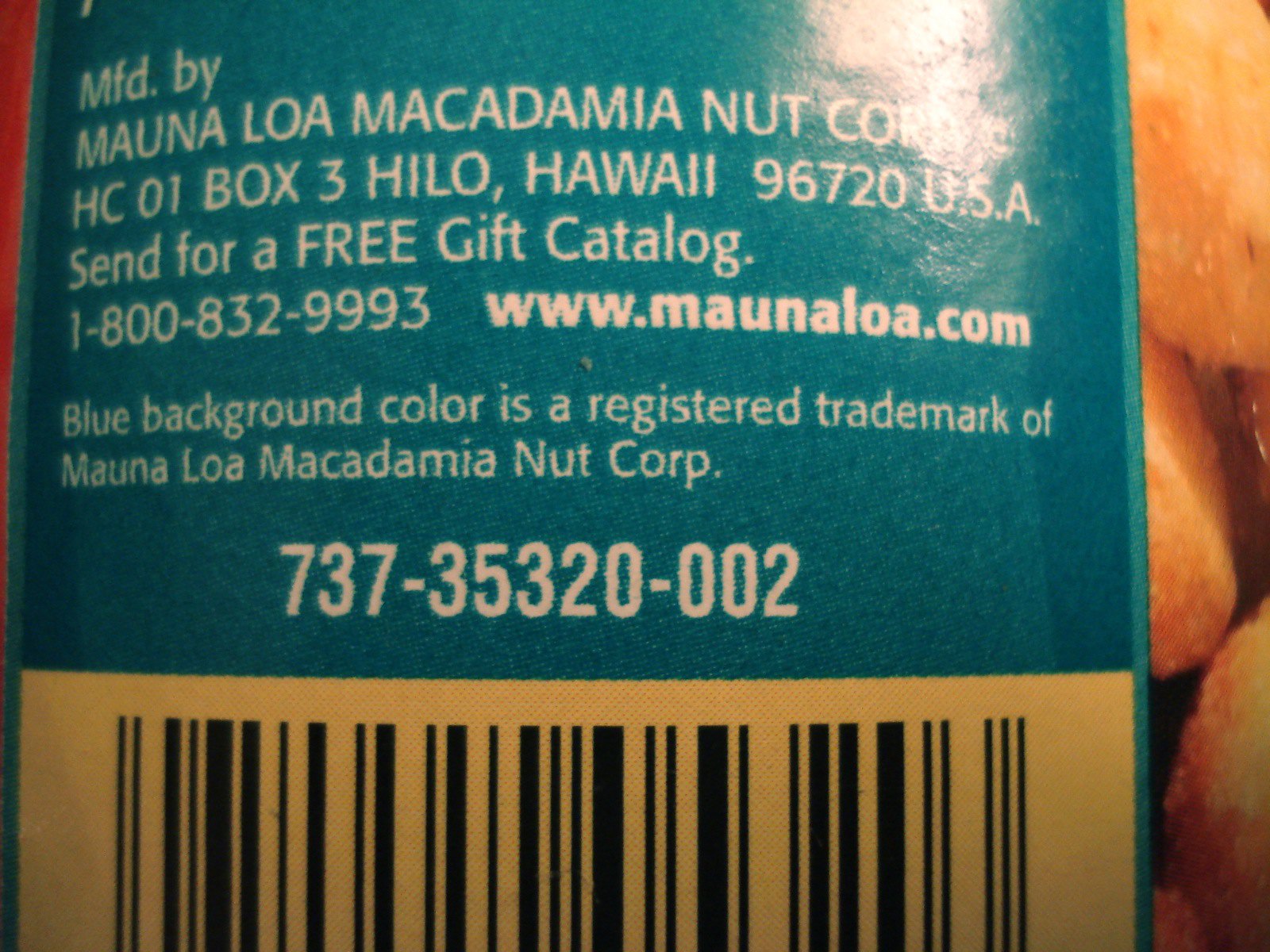This detailed close-up photograph captures the information label on a can of macadamia nuts. The label has a dark greenish-blue or turquoise background, which is stated to be a registered trademark of Mauna Loa Macadamia Nut Corp. Centered on the label in bold white text are the words "MFD. by," which stands for "manufactured by," followed by "Mauna Loa Macadamia Nut Company." The label includes the address HC-01 Box 3, Hilo, Hawaii 96720, USA. Below the address is an invitation to "Send for a FREE gift catalog" with a toll-free number, 1-800-832-9933, alongside the website address www.maunaloa.com. Beneath this information, there's a code, 737-35320-002, followed by a large barcode running horizontally across the label. The background also features images of macadamia nuts, reinforcing the product's identity. The detailed presentation and specific layout make it clear that this label belongs to a product from Mauna Loa Macadamia Nut Corp.